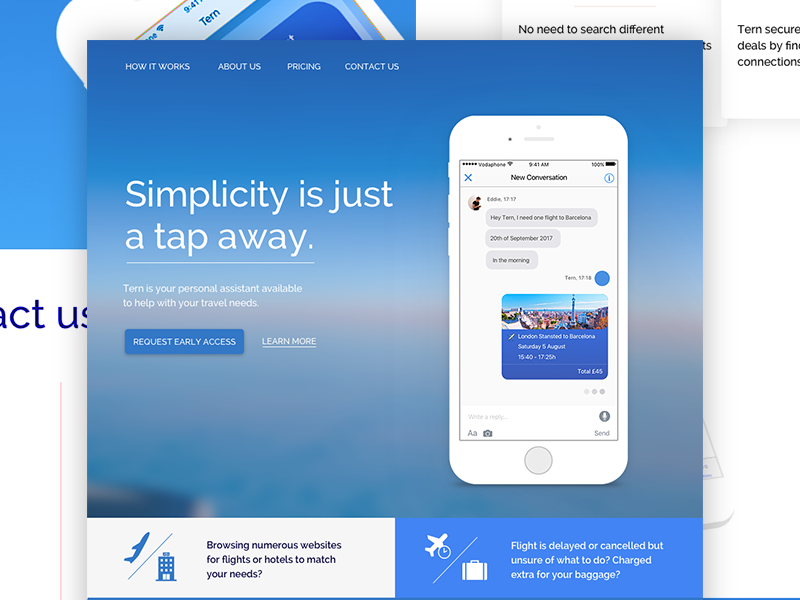The image is of a cell phone screen displaying an advertisement for an app named Tern, a personal assistant designed to assist with travel needs. The top part of the screen features an ad with the slogan "Simplicity is just a tap away." Below the slogan, the app's name, Tern (spelled T-E-R-N), is prominently displayed with the message: "Your personal assistant available to help with your travel needs." There are two options: a blue button labeled "Request Early Access" and a white button labeled "Learn More."

The screen also shows a simulated conversation within the app. A user message reads: "Hey Tern, I need one flight to Barcelona, 20th of September, 2017 in the morning." In response, Tern displays a flight option: "London to Barcelona, Saturday, August 5th," complete with departure and arrival times and a total cost of £45.

Above the chat, the app's navigation bar includes options such as 'How It Works,' 'About Us,' 'Pricing,' and 'Contact Us.' At the bottom of the screen, a blue box inquires, "Browsing numerous websites for flights or hotels to match your needs?" and asks in white text, "Flight is delayed or canceled but unsure of what to do? Charged extra for your baggage?"